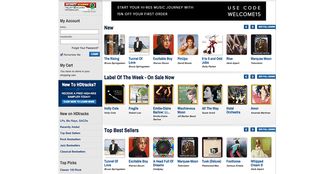A vibrant display of a music purchasing website interface is laid out with a clean and modern design. The top left corner prominently features a star icon, indicative of a premium or highlighted section. Below the star, a welcoming text and a user account section with options such as "Remember Me" are visible. Central to the interface is a vivid blue square that stands out, surrounded by seven rectangular images, each representing a different music piece categorized under "Top Best Sellers" and "Label of the Week – On Sale Now." The page is structured into columns on the left side, guiding the user through various sections of songs and albums, all detailed with accompanying images and descriptive text. The overall composition suggests a well-organized platform focusing on promoting popular and discounted music items.